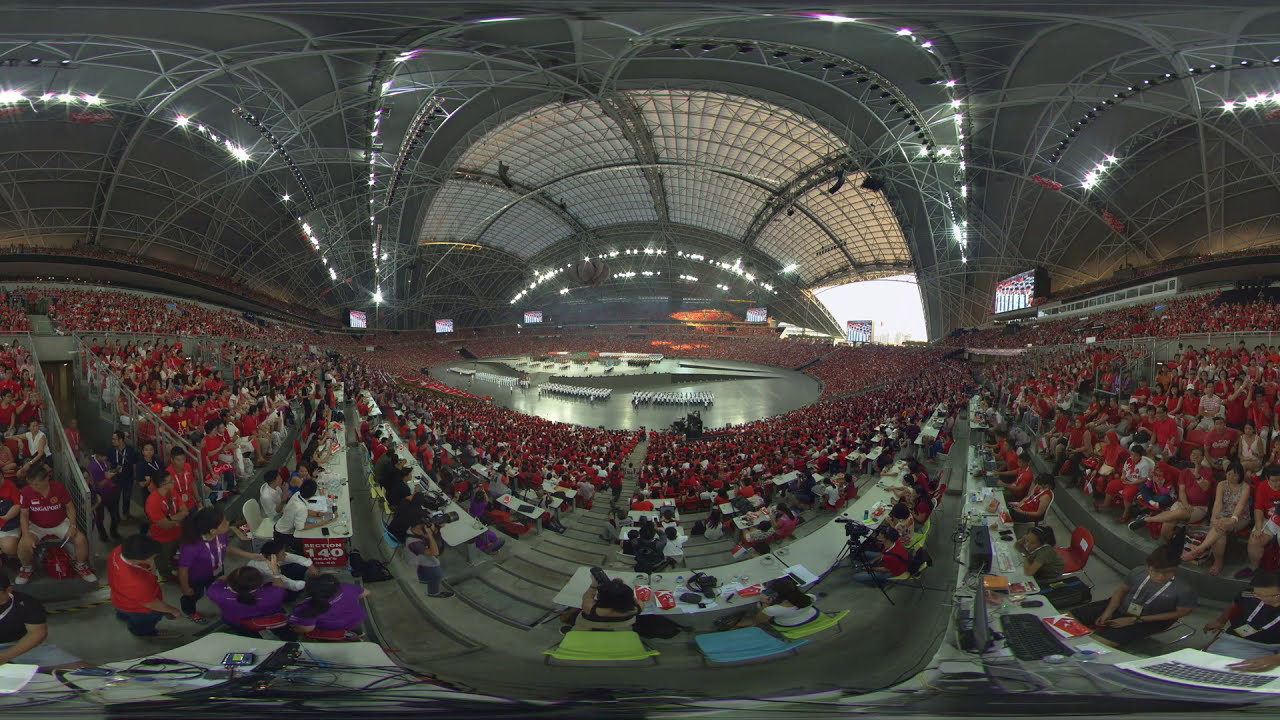Captured with a fisheye effect, the image showcases a grand indoor stadium with a prominent, curved, or domed roof, creating a distinctive warped perspective. The arena’s seating is mostly made of gray concrete, and it hosts a sea of spectators adorned in red T-shirts, suggesting a theme or supporting a home team. The stadium is flooded with natural light streaming through large windows in the dome above, highlighting the intricate steel framework supporting the roof.

At the center of the arena, a hard surface replaces any typical playing field, suggesting a setup for varied purposes such as a competitive event or a presentation. The area is equipped with ramps, hinting at a possible extreme sport event. Surrounding this central space, several judge’s tables and media desks are arranged, indicating preparations for either a broadcast or important evaluations during the event. The overall ambiance is one of anticipation and preparation, with every detail meticulously arranged to support the unfolding spectacle in this vast, dynamic space.